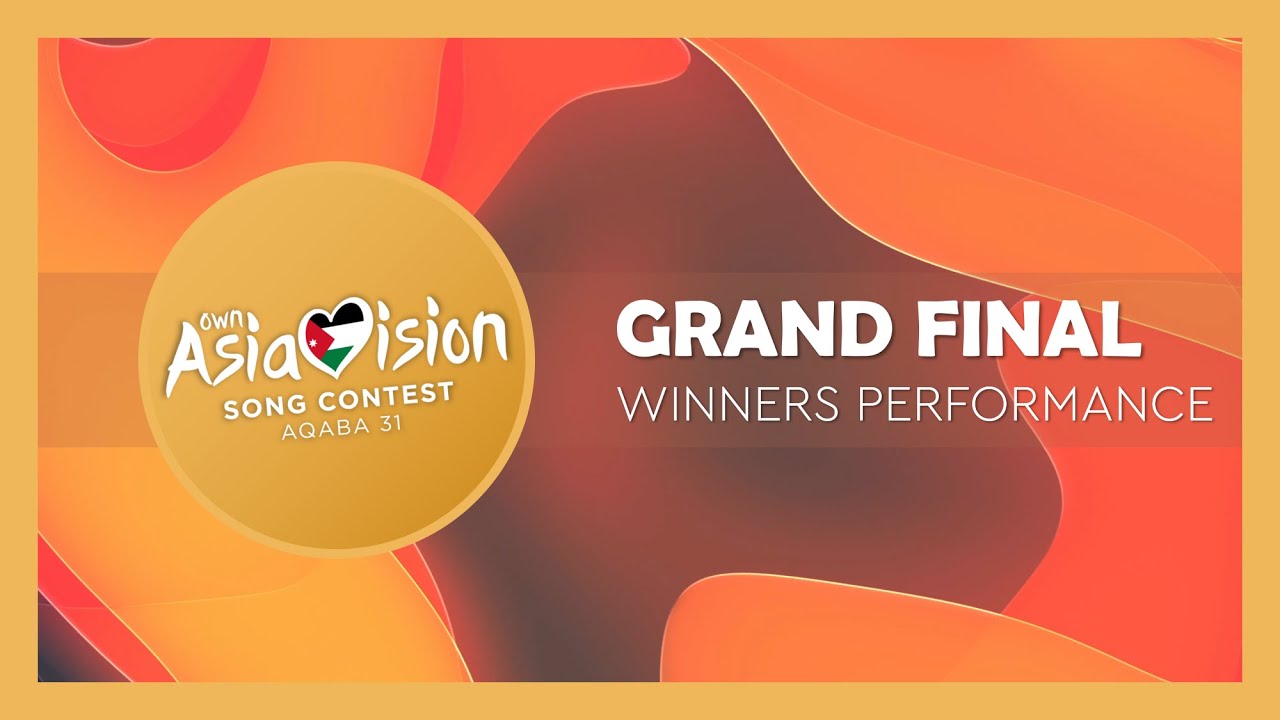This image captures an ad designed with vibrant details and an intricate layout. It features a dark mustard yellow border framing a rectangular space oriented horizontally. The background exhibits a blend of geometric areas in dark purple, orange, light orange, and even some brownish hues. Dominating the design, positioned on the left side is a gold or mustard yellow circle containing the text "Own Asia Vision Song Contest" with "AQABA 31" explicitly mentioned. Notably, the "V" in "Vision" is substituted with a heart shape adorned with black, green, and red decorations, indicative of a flag design. Adjacent to this, in white capital letters, it prominently announces "Grand Final" followed by "Winner's Performance" in a slightly less bold white font. This central strip cuts across the varying shades of orange and adds a cohesive element to the visual narrative. An orange frame further enhances the image's striking appearance.